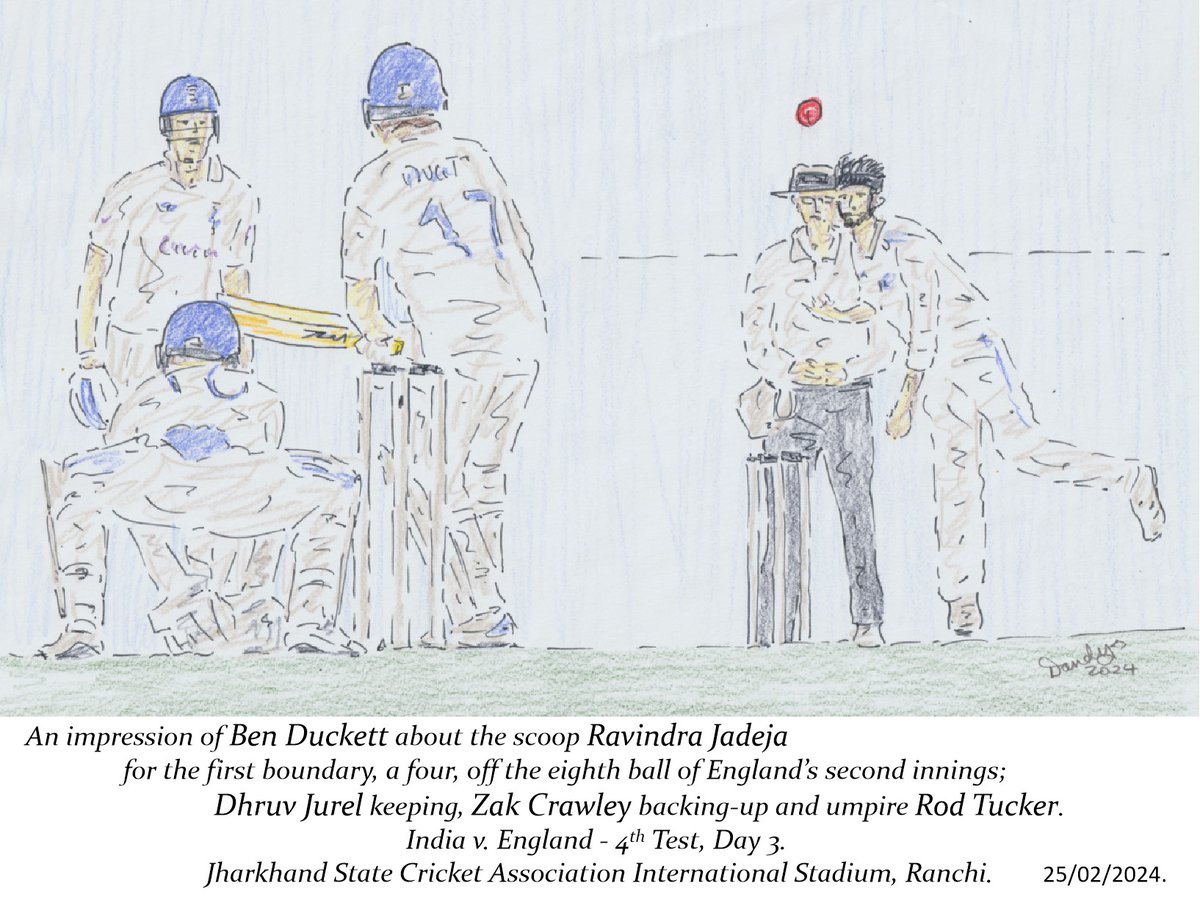This vibrant and detailed illustration captures a moment from a riveting cricket match at the Jharkhand State Cricket Association International Stadium in Ranchi. In the foreground, Ben Duckett is poised for a scoop shot, facing the first boundary off the eighth ball of England's second innings, delivered by Ravindra Jadeja. The red cricket ball is prominently visible, headed towards Duckett's bat. The scene includes four players, with Zach Crawley backing up and Dhruv Jhural keeping. Umpire Rod Tucker, distinguishable by his white and gray attire and fedora, stands in the background overseeing the play. The cricketers in white uniforms adorned with blue hats and numbers stand out against the light gray or light blue background, adding a dynamic contrast to the brown pitch. The image, rendered in a colorful blend of mediums resembling pen and colored pencil, is signed by the artist and dated 25-02-2024, encapsulating the intensity of the fourth test match, day three between India and England. The detailed depiction vividly brings to life the tension and excitement of this cricketing moment.